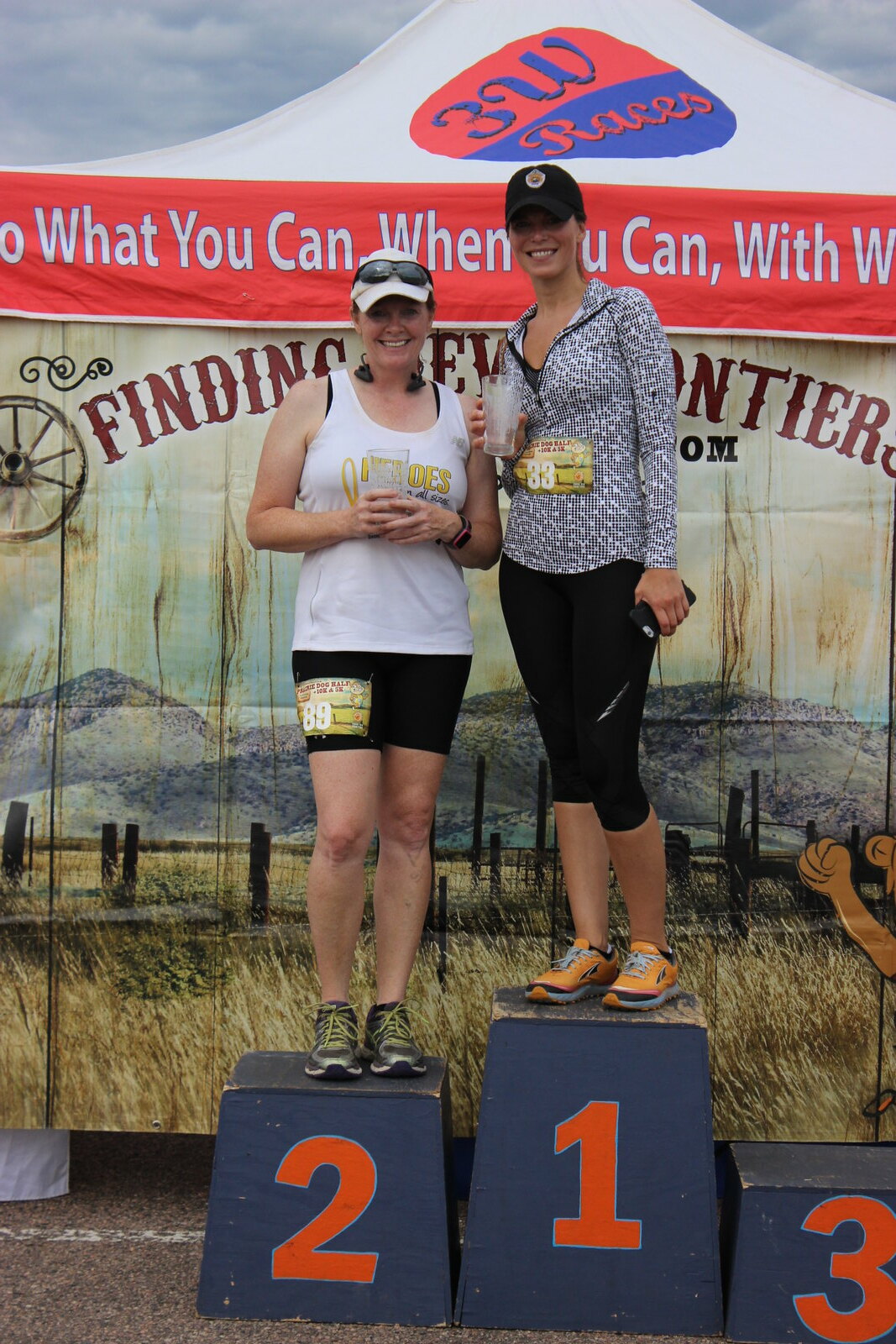This detailed, outdoor, daytime color photograph features two smiling Caucasian women in their mid-20s, standing on podiums after a race. The woman on the left, in second place, stands on a blue podium marked with a red number 2. She sports a white tank top with yellow print, black bicycle shorts, running shoes, a white baseball cap with sunglasses resting on the bill, and headphones around her neck. Her race number, 89, is displayed on a banner attached to her shorts. The first-place woman is to her right, standing on a slightly taller, dark blue podium marked with a red number 1. She wears a black baseball cap, a light gray long-sleeved zip-up top, black pants, and orange shoes. Her race number, 33, is visible on her top. Both women are holding clear glasses, presumably of water, and smiling at the camera. Above them is a large white canopy tent with "3W Races" printed on it. A red banner below the canopy reads, "What You Can, When You Can, With," but the rest is cut off. Behind them, a backdrop banner depicts grass and mountains with a red-lettered slogan that is partially obscured but includes the phrase "Finding New Frontiers." There is also a blue podium with the number 3 to the right and below the women. The sky visible above the canopy is cloudy blue, enhancing the outdoor setting.